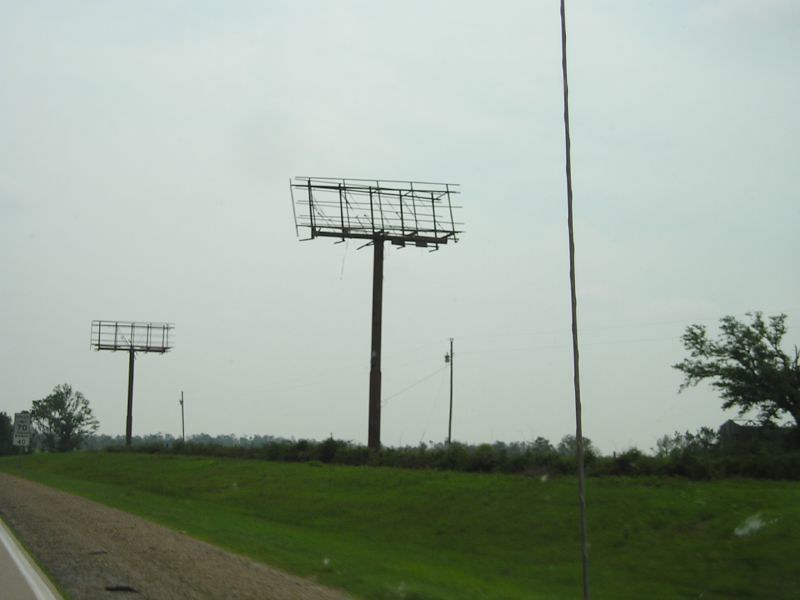The image depicts a semi-rural landscape marked by two large, empty billboard structures standing prominently against an overcast sky. The towering billboards, stripped of their advertisements, expose their skeletal frameworks, lending a sense of abandonment and desolation to the scene. The sky is cast in shades of gray, further accentuating the gloomy ambiance. The flat terrain is dotted with patches of green grass and a smattering of trees in the background, hinting at the area's sparse vegetation. A road sign displaying a speed limit of 70 miles per hour suggests the proximity of a major highway or thoroughfare. A utility pole positioned on the right side of the image intersects the frame vertically, creating a stark contrast with the horizon and the road's horizontal lines, adding a dynamic element to the composition.